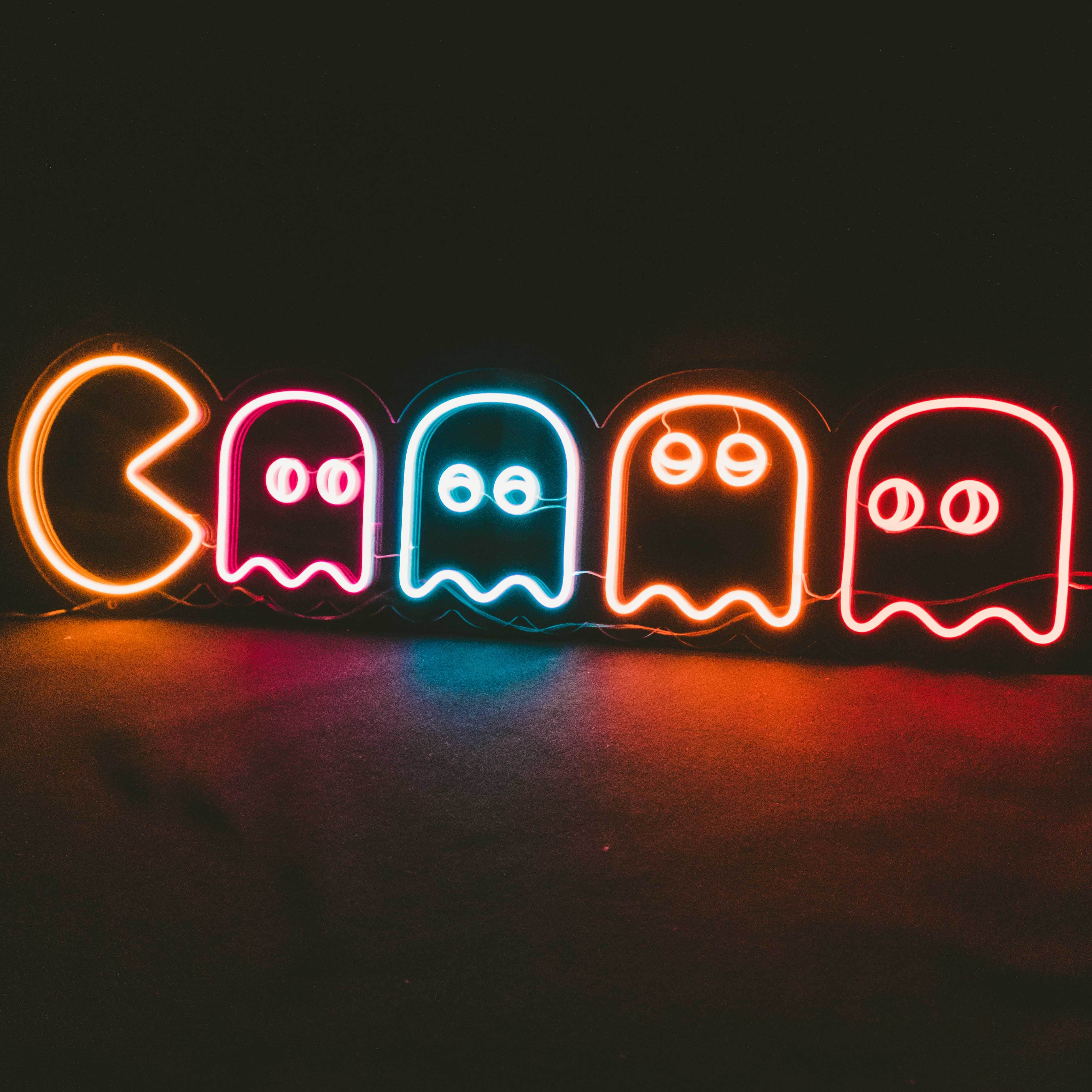This photograph captures a vivid neon or LED art installation depicting characters from the classic video game Pac-Man. At the center of this dark composition is Pac-Man, illuminated in yellow, positioned on the left side, appearing poised to gobble up the four ghosts arranged to his right. The ghosts, each rendered in distinct vibrant colors—pink, blue, orange, and red—are spaced evenly, with their eyes gazing in various directions: the pink ghost looks to the right, the blue ghost looks down, the orange ghost looks up, and the red ghost looks to the left. The dark background enhances the glow of the lights, which cast colorful reflections on the floor below, creating a striking rainbow effect. Behind the installation, an intricate web of wires can be seen, suggesting the technical setup involved in making this dynamic display come to life.